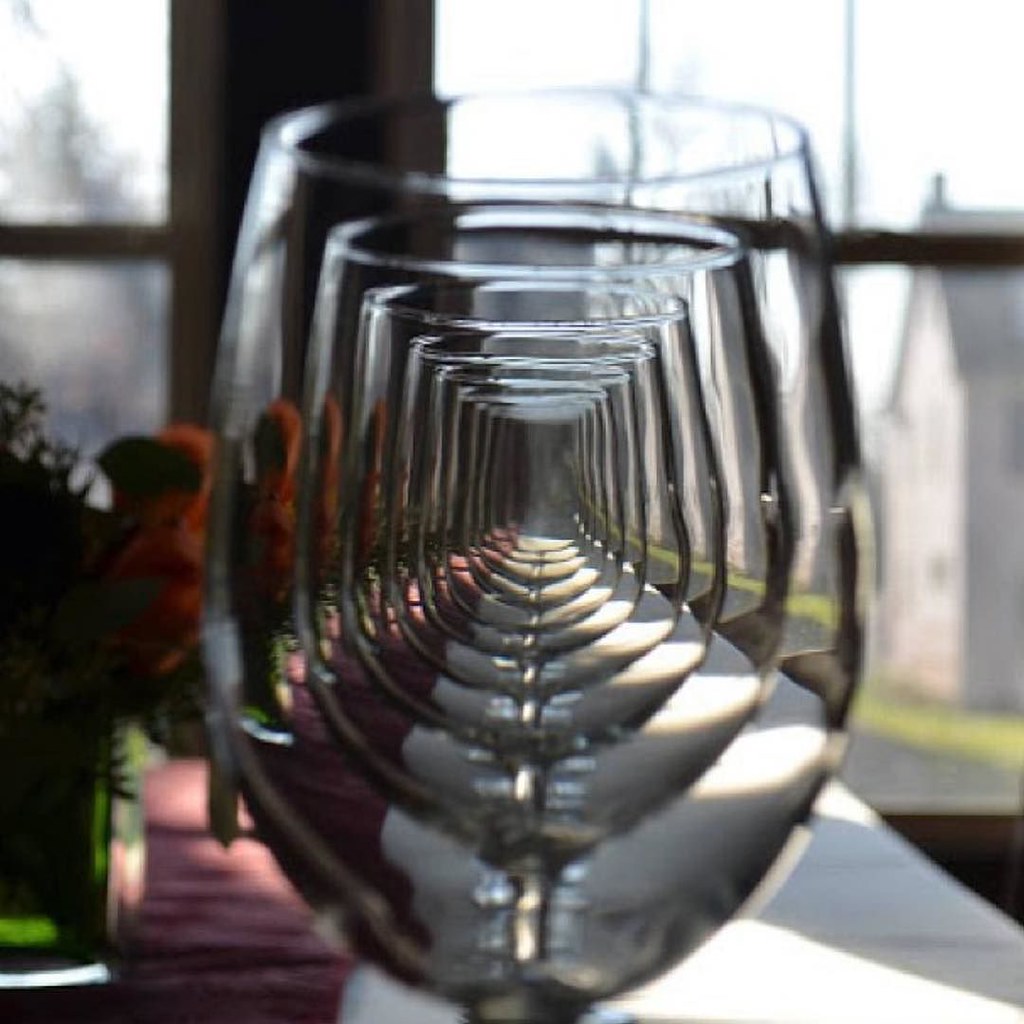This photograph captures a mesmerizing row of twelve identical wine glasses, each perfectly lined up to create an illusion of an infinite hallway as you peer through them from the front to the back. The symmetry and parallel alignment of the glasses cast a reflective and repetitive pattern across a white table that is partially cloaked in shadow, suggesting the presence of sunlight. To the left of the wine glasses, dark green vases hold vibrant red roses, adding a splash of color against a dark red placemat. The background reveals an out-of-focus scene of a house and its chimney, visible on the right side of the image through transparent window panes, enhancing the overall depth and complexity of the composition.